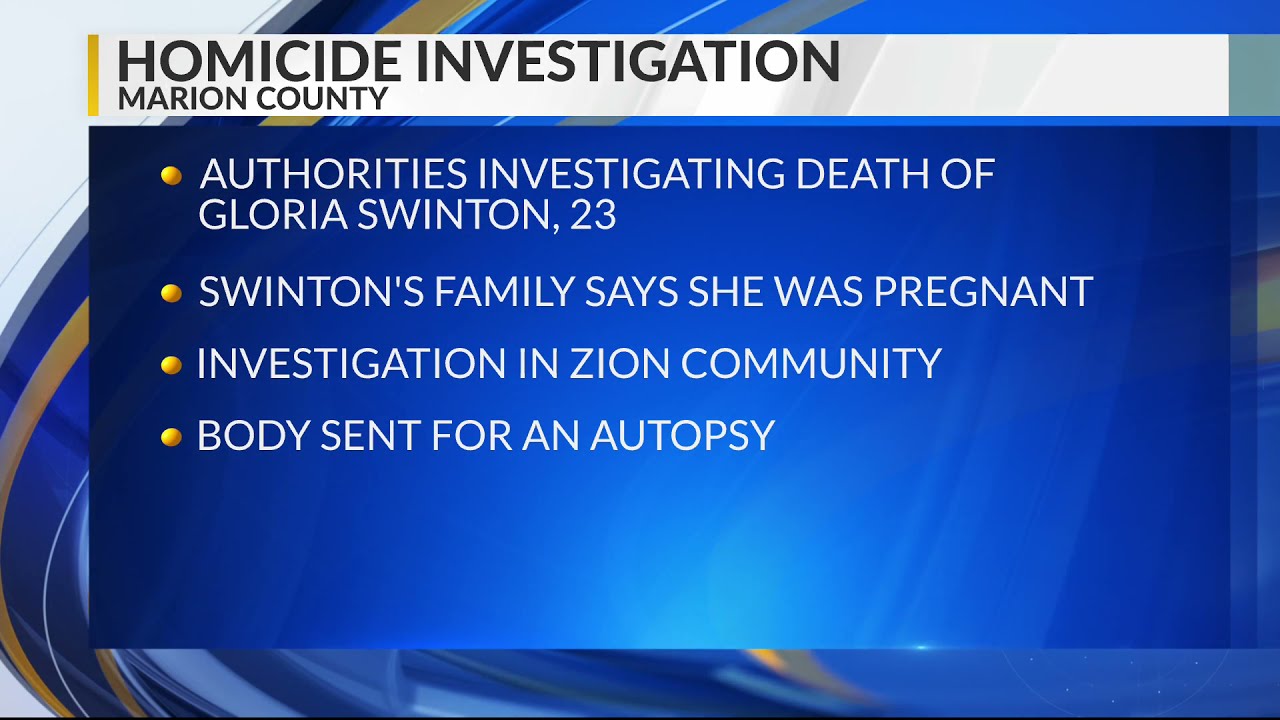This still frame from a high-resolution news broadcast captures the somber details of a developing story. The background features a dynamic, swirling pattern with colors ranging from white in the top left, transitioning to gray, dark blue, gold, and then back to blue and gray, creating a whirlpool-like effect. At the top of the screen, a slim vertical white box with bold black font announces, "Homicide Investigation, Marion County." Below this, a prominent blue box with four yellow bullet points presents the critical details in white text: "Authorities Investigating Death of Gloria Swinton, 23," "Swinton's family says she was pregnant," "Investigation in Zion Community," and "Body sent for an autopsy." The meticulously structured graphic, with its bold and clear typography, conveys the gravity and emerging details of this homicide investigation.